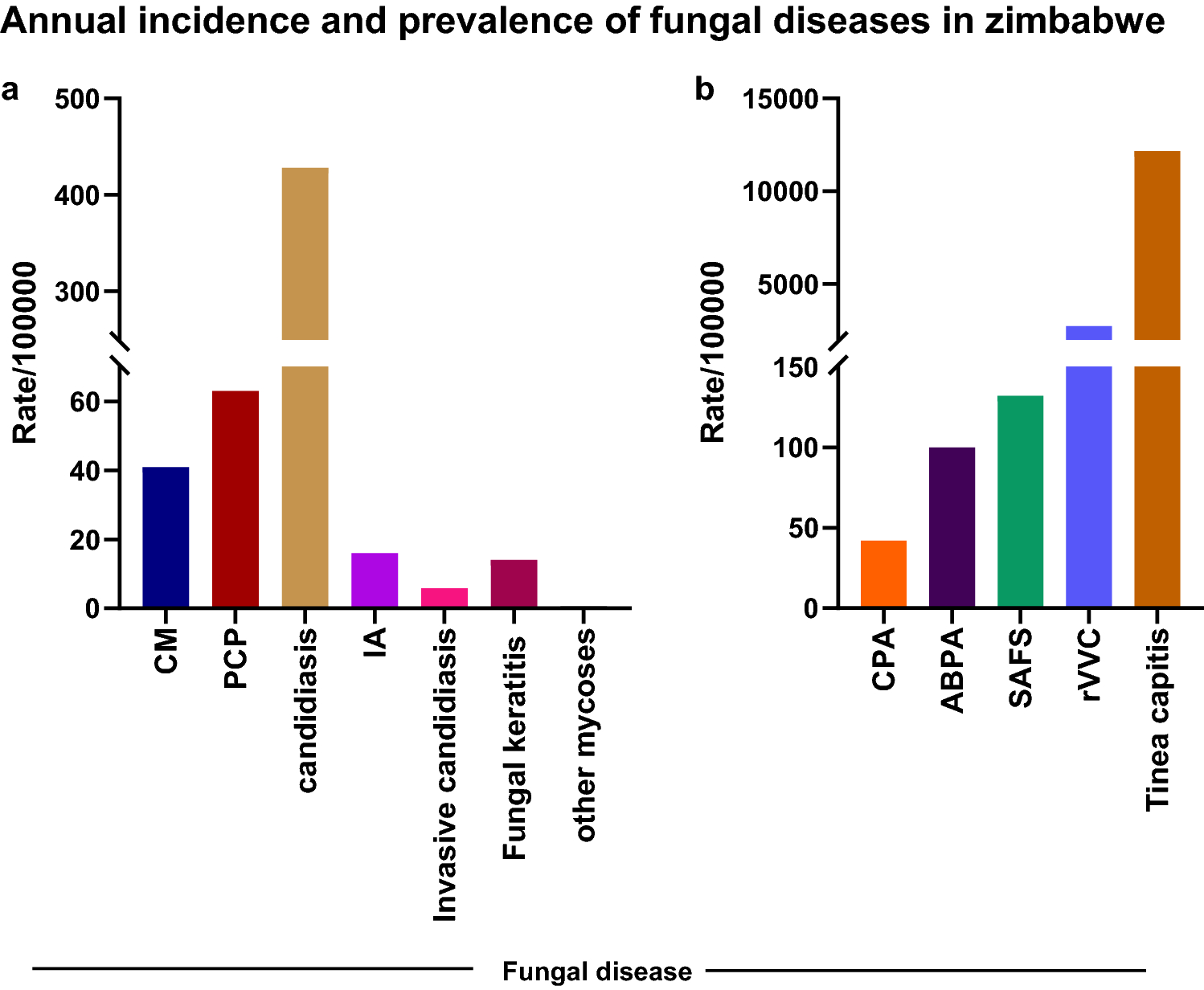This digital informational piece presents comprehensive data on the annual incidence and prevalence of various fungal diseases in Zimbabwe, an African country. The title, "Annual Incidence and Prevalence of Fungal Diseases in Zimbabwe," is prominently displayed at the top in black text. The piece features two detailed bar charts, each illustrating the rate per 100,000 population for different fungal diseases.

The chart on the left categorizes diseases along the x-axis with the y-axis representing the rate per 100,000. The largest bar, colored brown, signifies the highest incidence rate for condidius. Other diseases such as CM, PCP, candidiasis, invasive candidiasis, CPA, and SAFS are also represented with different colored bars.

The right-hand chart also displays rates per 100,000 for additional fungal diseases, highlighting tinea capitis as having the largest incidence with varied colors distinguishing each disease. Abbreviations such as RVVC, IA, and fungal keratitis are employed to denote specific diseases.

This datagraphic employs a variety of colors including tan, brown, maroon, blue, green, dark blue, purple, and pink to differentiate between the various disease rates, making the information visually accessible and straightforward. The precision and thoroughness of the data visualization underscore the critical health insights about fungal disease prevalence in Zimbabwe.